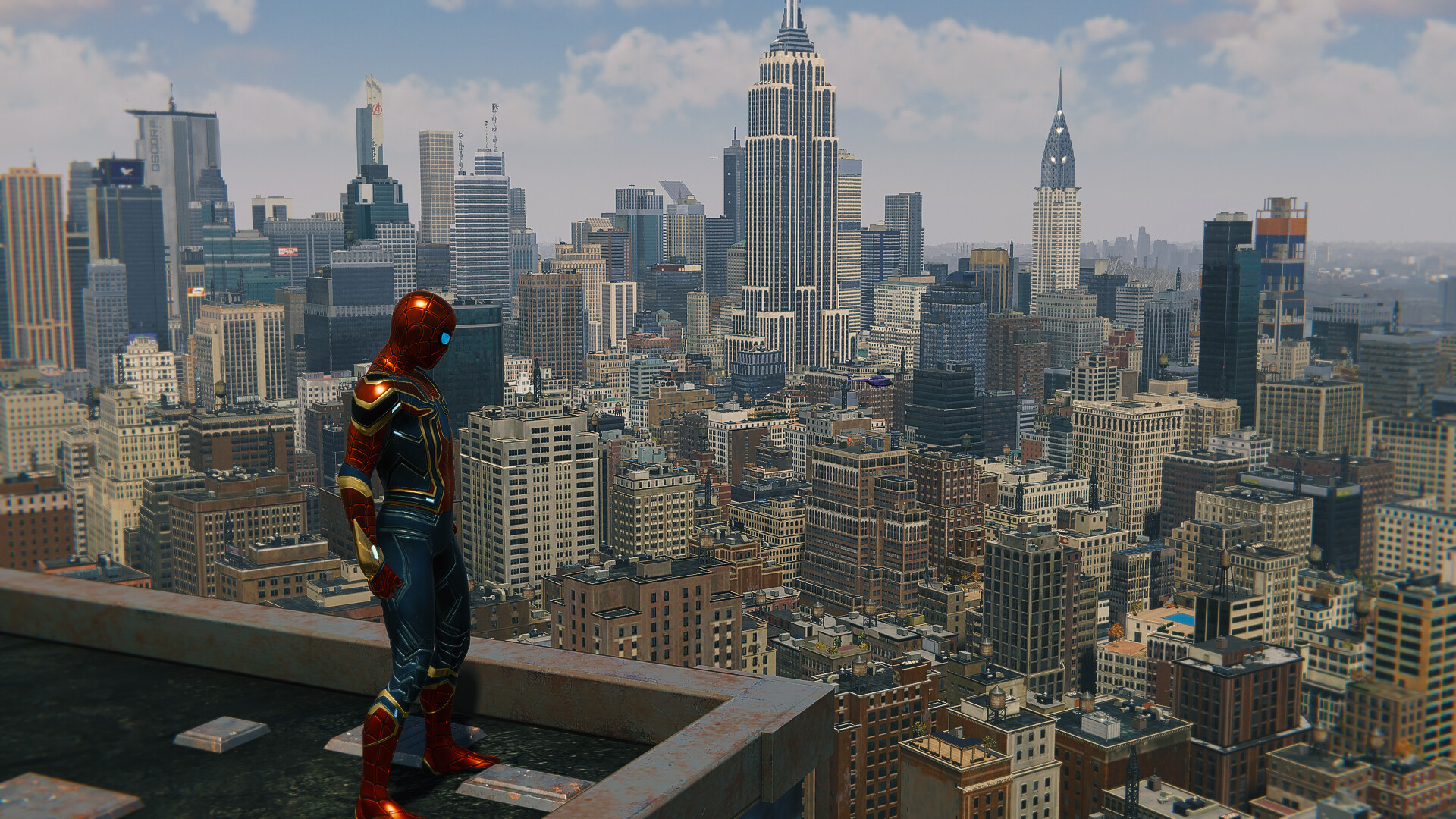An intricately designed image portrays a bustling city skyline that bears a striking resemblance to New York City, though subtle details suggest it may be a digitally created or fictional metropolis. The skyline features an array of high-rise buildings sprawled beneath a bright midday sky adorned with fluffy clouds and a hint of smog. To the left side of the image, a partial view of a building in the foreground reveals a striking figure standing on the edge – a costumed superhero with a visually captivating suit.

The superhero's helmet has a red metallic sheen, reminiscent of Spider-Man's iconic mask, complete with blue eye elements shaped similarly to those of Spider-Man. The suit itself is an innovative blend of Iron Man and Spider-Man aesthetics; it features a mix of gold and red metallic accents interwoven with vivid red, black, and blue components. The form-fitting bottoms and legs of the suit display a blue metallic hue, while the arms are adorned with an interplay of red, black, and gold. The boots gleam in a solid red metallic tone. This enigmatic figure stands stoically, gazing down protectively over the cityscape below.